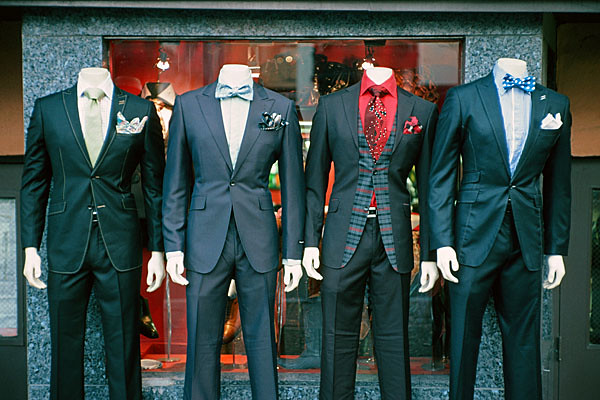In this photograph, we see four headless male mannequins lined up in front of a store display window. Each mannequin is dressed in a formal suit, exhibiting a variety of styles and colors. The mannequins are positioned outside the store, against a backdrop of a large glass window framed by dark gray marble flecked with white and brown specks. The interior of the display window features red felt and red walls, adding a rich contrast.

From left to right, the first mannequin is dressed in a black suit paired with an olive green tie, a white undershirt, and a white, blue, and pink corsage in the right pocket, wearing black dress pants. The second mannequin stands out with its dark blue tuxedo, complemented by a light blue bow tie, a dark blue and tan corsage, and a white dress shirt, alongside dark gray or black pants. The third mannequin features a black tuxedo with dark blue, dark gray, and red plaid accents, a red undershirt, a tie that is half maroon and half red with small white and black squares, a maroon corsage with black and white details, and black dress pants. Lastly, the fourth mannequin showcases a black tuxedo, black dress pants, a light blue undershirt, a dark blue bow tie with white polka dots, and a white corsage in the right pocket.

Together, these mannequins create a striking display of elegant formal wear in front of the chic and sophisticated storefront.